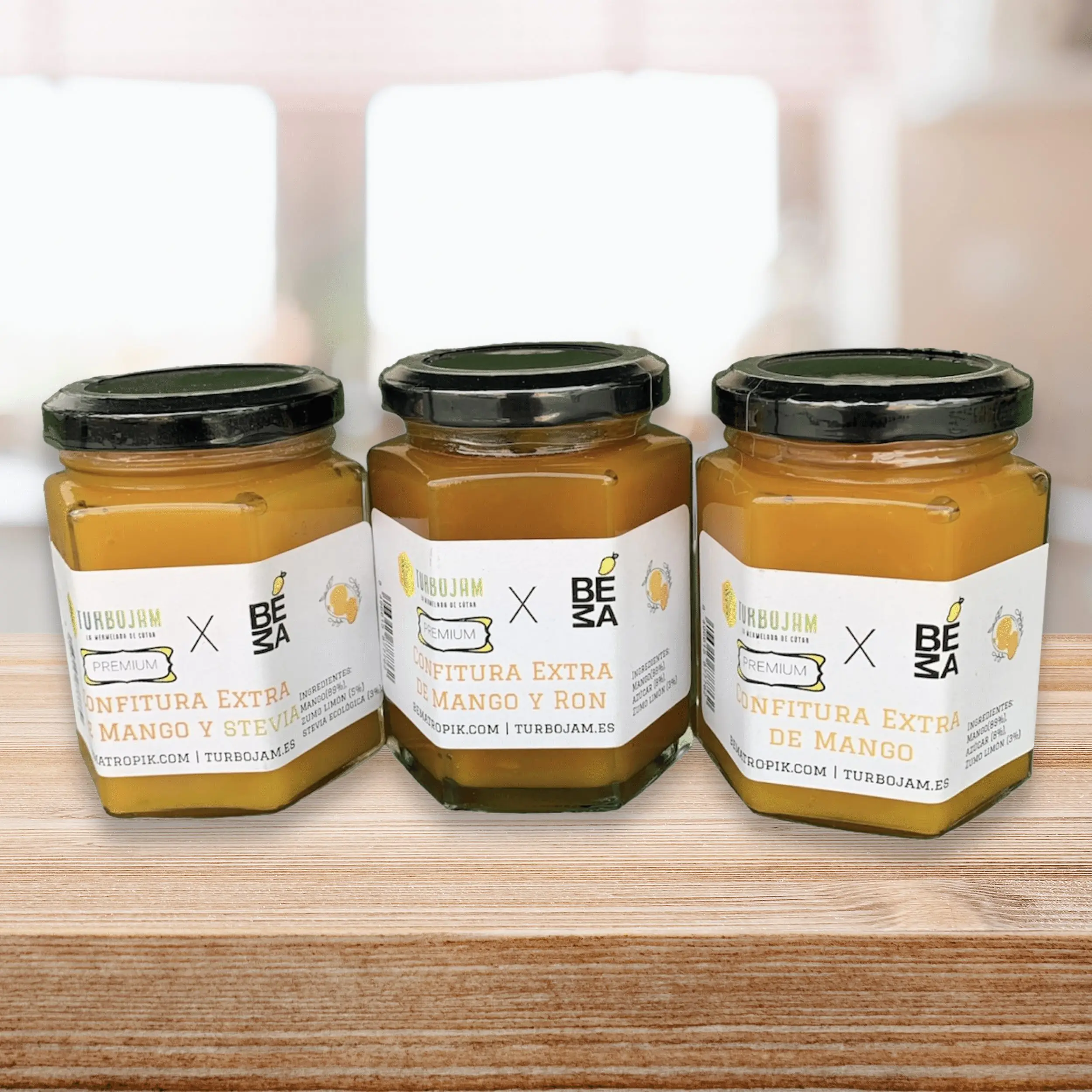This rectangular close-up product photo showcases three hexagonal glass jars with shiny black lids, neatly arranged next to each other on a thick, light wooden shelf. The jars, which are in focus against a blurred background, each contain a yellowish-brown substance resembling various types of mango jelly or sauce. The jars feature white labels displaying the company logo, BEAM, and the product name, TurboJam. The labels also indicate the specific types of jam: one is "mango y Ron," another is "mango y Stevia," and the third simply "mango." The middle jar's contents appear slightly darker than the other two. All three products, despite minor variations in color, underscore the premium quality and diverse flavors of the brand's mango confitura offerings.